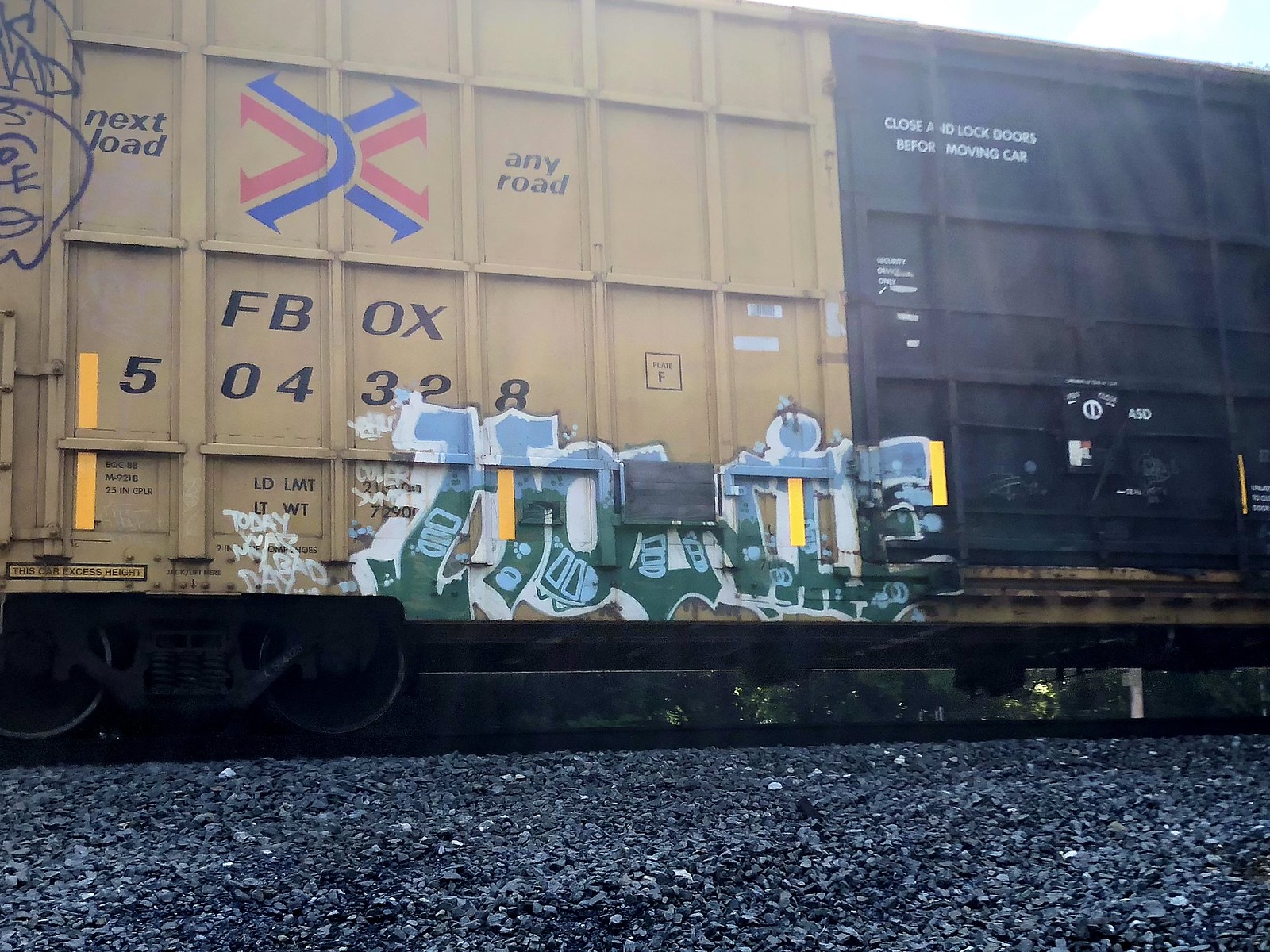This color photograph, taken outdoors in a train yard, captures the side of two freight train cars against a dark gray and black gravel ground. The train cars are positioned on railroad tracks, with the car on the left being tan and the one on the right being black. Both cars display commercial writing, with the tan car notably marked with "Next Load Any Road" alongside the identifiers "FBOX 504328" and an emblem featuring interlocking blue and red X's with notches at the ends.

The black car bears the instruction "Close and lock doors before moving car" in small white writing. Each car is adorned with graffiti, predominantly on the tan car, displaying varied colors like blue, light blue, green, yellow, and white. The graffiti includes phrases such as "Today was my bad day," amidst other illegible words and abstract designs, adding a layer of urban artistry to the industrial scene. The gravel around the train tracks further emphasizes the rugged, outdoor environment of the train yard.